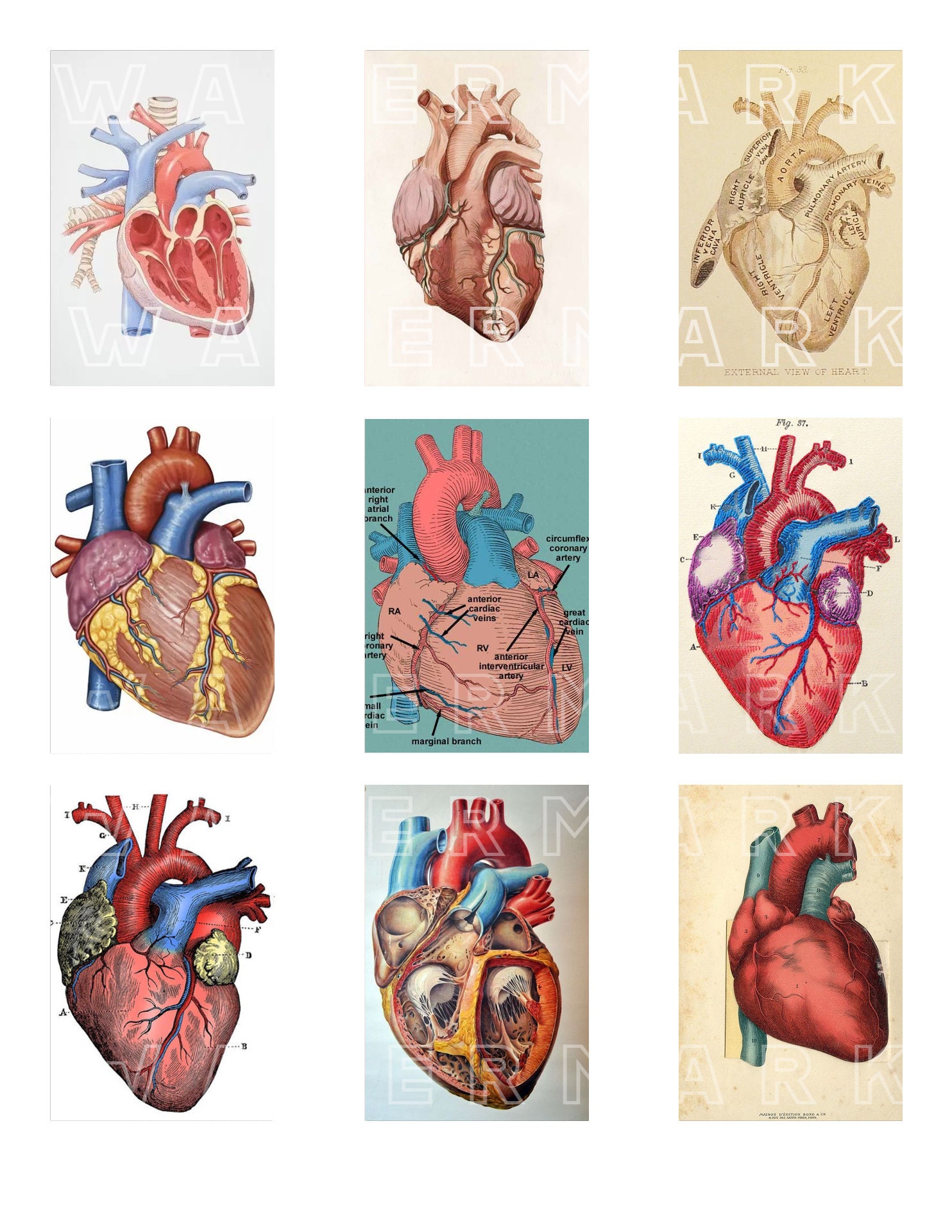The image displays a 3x3 grid of nine distinct illustrations of the human heart, arranged in three rows and three columns. Each square or rectangle in the grid contains a detailed rendering of the heart, varying in style, complexity, and color scheme. Some illustrations are modern, while others appear historical, suggesting a range of eras or artistic interpretations. Most of the hearts feature anatomically accurate details, including visible veins and arteries, and some are cutaway views revealing internal structures like ventricles. The backgrounds differ: a few are white, one is sepia-toned, and another uses faded colors. Several images include fine print labeling various parts of the heart, indicative of their use as educational tools, possibly for medical students. Across the entirety of the grid, block-letter text reading "watermark" is superimposed horizontally in multiple locations. The middle image seems to be more detailed with annotations that are too small to read, hinting at a scholarly or instructional context. Vibrant reds, blues, and greens dominate most illustrations, though one heart is depicted in tan, adding to the visual diversity.